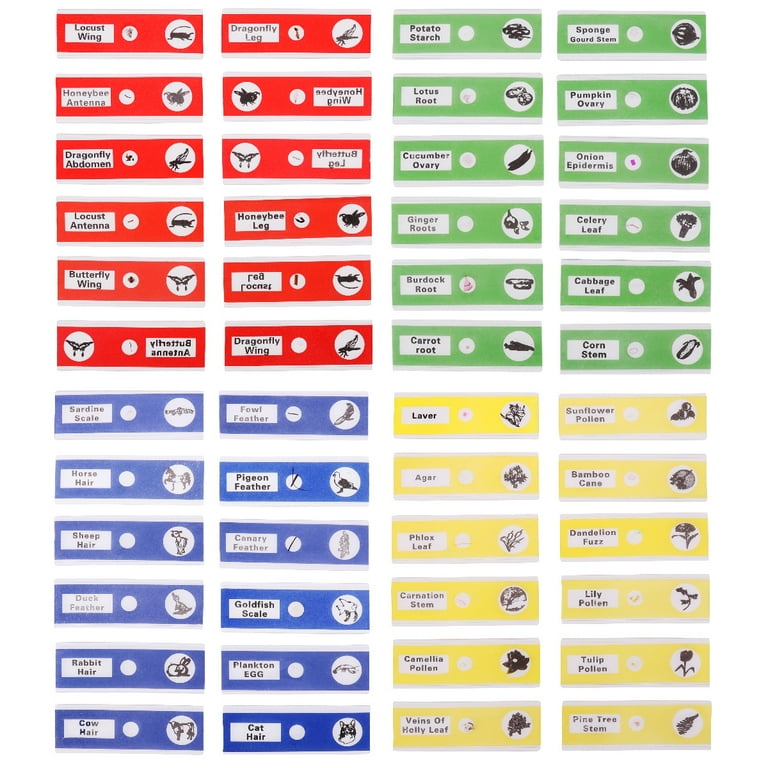The image consists of a composite photograph showcasing detailed identification labels, meticulously arranged in four colored quadrants. The upper left quadrant features six red blocks, each highlighting different insect parts such as locust wings and honeybee antennae, accompanied by text descriptions and illustrative drawings of the insects. The upper right quadrant contains six green blocks dedicated to different components of vegetables, resembling gardening labels with close-ups and detailed descriptions of items like potato starch. The lower left quadrant displays six blue banners focused on various animal parts, each providing a textual explanation and a detailed visual of the animal from which the part is derived. Finally, the lower right quadrant encompasses six yellow banners, each elucidating different components of flowering plants, complete with descriptive text and close-up imagery. Each label within the quadrants effectively combines textual information with visual aids to enhance the identification and understanding of insects, vegetables, animals, and flowering plants.